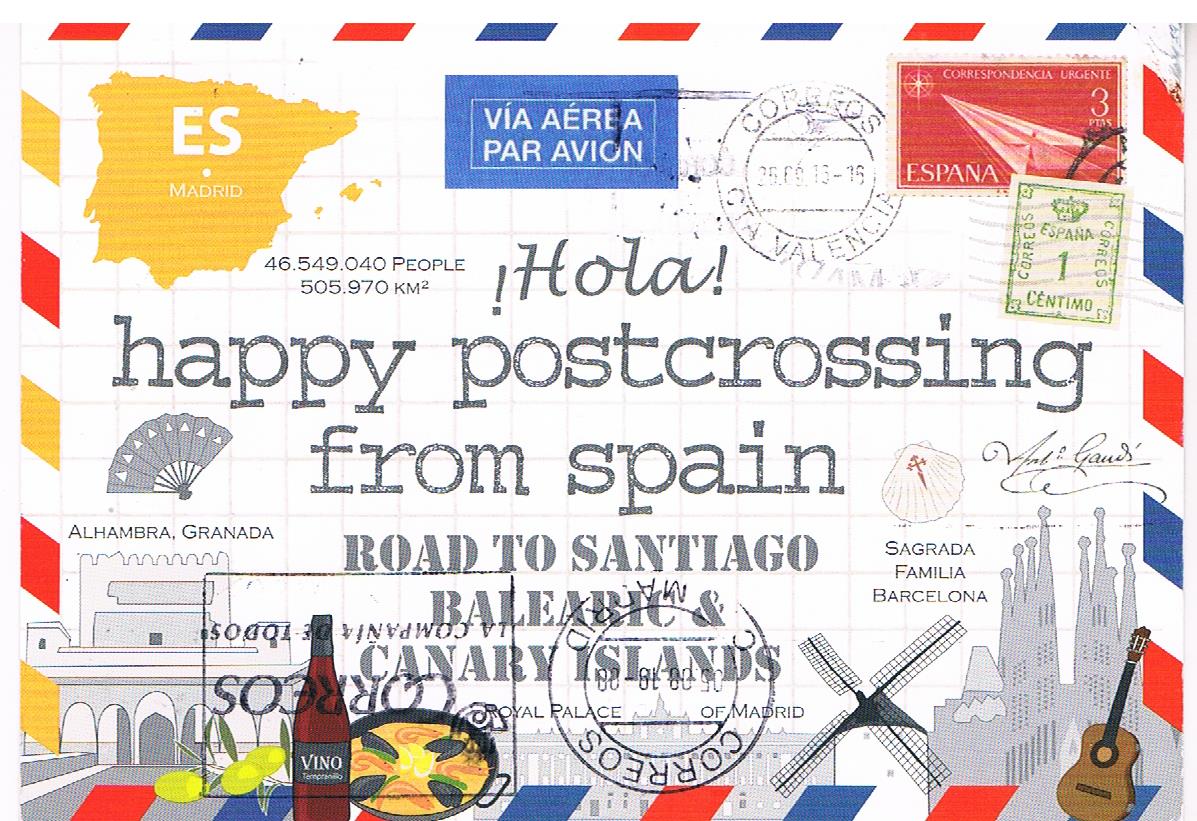This digitally rendered postcard is bursting with vibrant, multicolored elements and artistic touches, making it a captivating visual treat. The image is framed with a lively border featuring alternating rhombuses in red, blue, and yellow, and stripes in red, blue, and yellow, adding to its dynamic appearance. Prominently featuring various objects and text, the postcard showcases stamps, bottles, food items, guitars, and depictions of buildings. In the top left corner, a yellow map of Spain labeled "ES Madrid" stands out, while a blue box with "Via Herrera Par Avion" and a red rectangle bearing the number three in white text ("Espana") add further detail. The center of the postcard bears the cheerful message, "Hola, Happy Post Crossing from Spain. Road to Santiago, Balearic Islands, and Canary Islands." 

Scattered across the postcard are diverse stamps and artistic sketches, including yellow olives, a wine bottle, a paella pan, a detailed windmill, a cityscape in gray, and a guitar in the bottom right corner. In addition, a small seashell labeled "Sagrada Familia Barcelona" and a beer bottle appear in the bottom left. The background predominantly features a white color, enhancing the vivid colors and intricate details that adorn the postcard. The overall impression is one of a meticulously crafted, visually rich celebration of Spanish culture and landmarks.